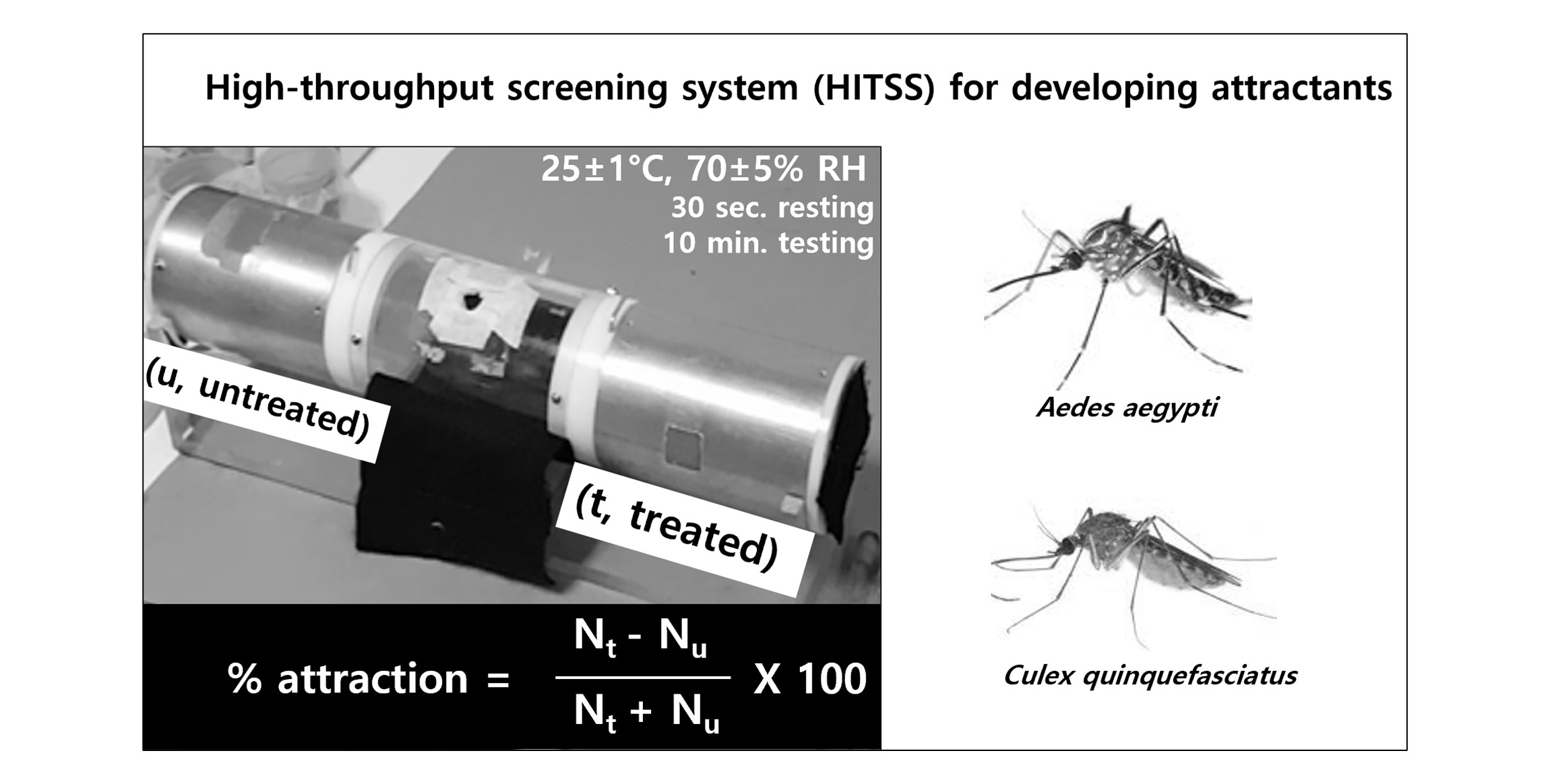This is a detailed scientific infographic bordered in black, with a white rectangular centerpiece featuring both text and images. The heading reads "High-Throughput Screening System (HITSS) for Developing Attractants." Emphasizing technical details, the infographic includes two black-and-white images of mosquito species on the right, labeled "Aedes aegypti" and "Culex quinquefasciatus." On the left, a metallic cylindrical device is depicted, denoted with "U untreated" and "T treated" on either end. Below this device, key environmental conditions are listed as "25 ± 1 degree Celsius, 70 ± 5 percent RH, 30 seconds resting, 10 minutes testing." An equation at the bottom reads: "Percent attraction = (NT - NU) / (NT + NU) × 100."